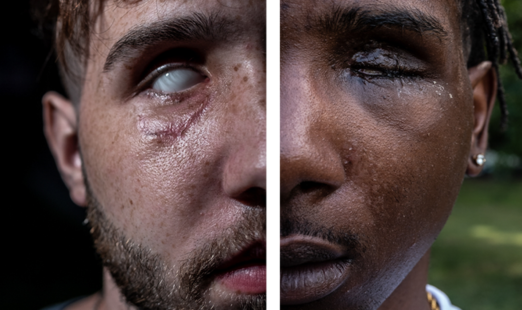The image is a composite of two distinct photographs placed side by side, separated by a white stripe down the middle. On the left, the close-up shows a man's face with a full beard and mustache; he has completely white eyes with no visible pupils or irises. This image has a solid black background, enhancing the eerie appearance of his eye. His hair is dark, and he seems to be wearing a dark-colored shirt, possibly blue or black. On the right, another close-up shows the right half of a man's face. He has a thin mustache, brown dreadlocks, a jewel stud earring in his ear, and his eyes are closed. He appears to be wearing a white collared shirt, and the background is a blurry, out-of-focus grassy area. Together, these images create a striking and surreal contrast between the two faces, but they do not appear to be of the same person.